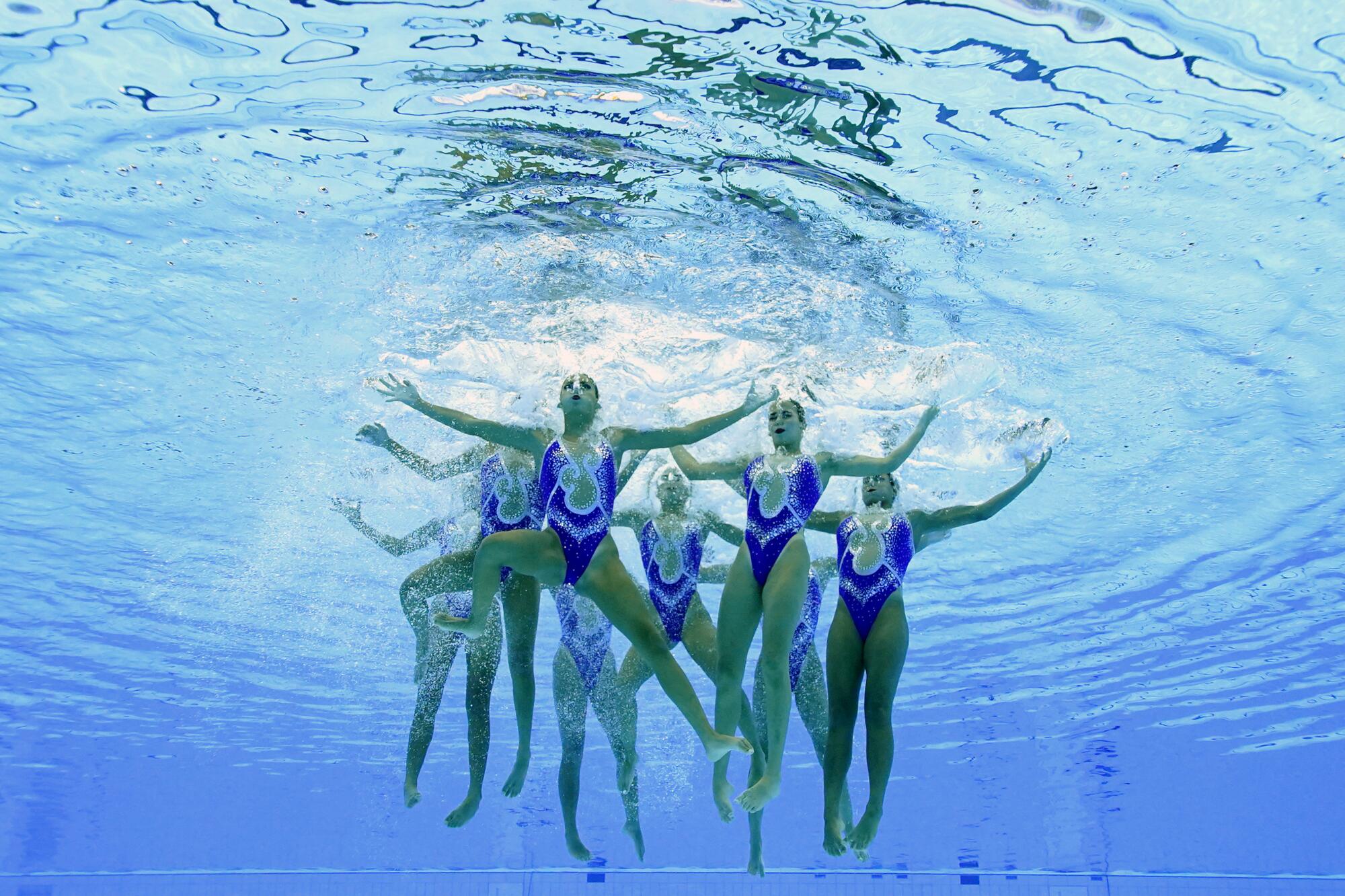This underwater photograph captures a team of seven to eight young female synchronized swimmers, clad in matching blue one-piece performance swimsuits accented with intricate silver, white, and occasionally gold designs. The swimsuits are notably detailed, featuring a teardrop shape in the center and sparkly V and U patterns. The swimmers are submerged in crystal-clear, light blue water of what appears to be an Olympic-sized swimming pool. They are clustered in a circle formation, holding their arms outstretched and slightly bent at the elbows, creating graceful lines in the water. Some have their legs perfectly straight, while others exhibit varied poses with bent knees or elevated legs, suggesting the start of an underwater routine. Bubbles escaping from their mouths, closed eyes, and peaceful expressions add to the serene yet dynamic atmosphere. The photograph, taken from below looking upwards, captures the ripple effects, foamy splashes, and glimmering light filtering through the water's surface, underscoring the beauty and precision of their synchronized performance.